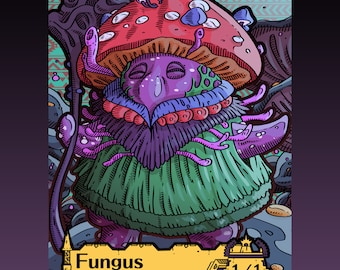The image is a digital art token with a square format featuring a vividly colored small rectangular scene. The image width is approximately two inches and the height is around an inch and a half. This scene is framed by quarter-inch wide borders on each side that transition from black at the top to a deep purple at the bottom. 

At the center is a whimsical, purple humanoid creature, resembling a fungus, with stubby, tentacle-like arms and short legs. The creature is adorned with a layered green coat with red circular accessories at the top and a blue collar. It has a closed-eyed, content expression on its purple face, highlighted by a thick, bulbous nose. Small green markings are visible on the creature's left side.

The head of the creature is topped with a mushroom cap hat that is domed and red with white spots and a brown underside. Two purple antennae protrude from the top of the hat. Below its thick nose, the creature sports a triangular-shaped gray beard with purple objects growing out from the edges and a blue line featuring red circular objects beneath it. 

In one of its arms, it grasps what appears to be a long wooden staff, although in some interpretations, it appears as a purple staff. The creature stands on a raised yellow area, and beneath this platform, the word "fungus" is printed in black. The overall background design includes a swirly, funky pattern, enhancing the playful, video game-like aesthetic of the piece.